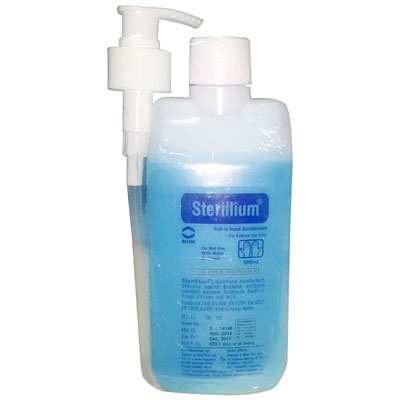The image showcases a clear plastic bottle filled with blue liquid, prominently centered on a completely white background. The bottle features a white cap on top, and attached to its left side is a pump mechanism with a long clear tube and a white nozzle, appearing as an accessory. The label on the front of the bottle, a blue rectangular shape, prominently displays the brand name "Sterillium," believed to be a type of hand sanitizer, although the remaining text is too small to read. The photograph's simplistic and bright setup suggests it was taken in a lightbox, likely intended for use on a website where the product is sold.